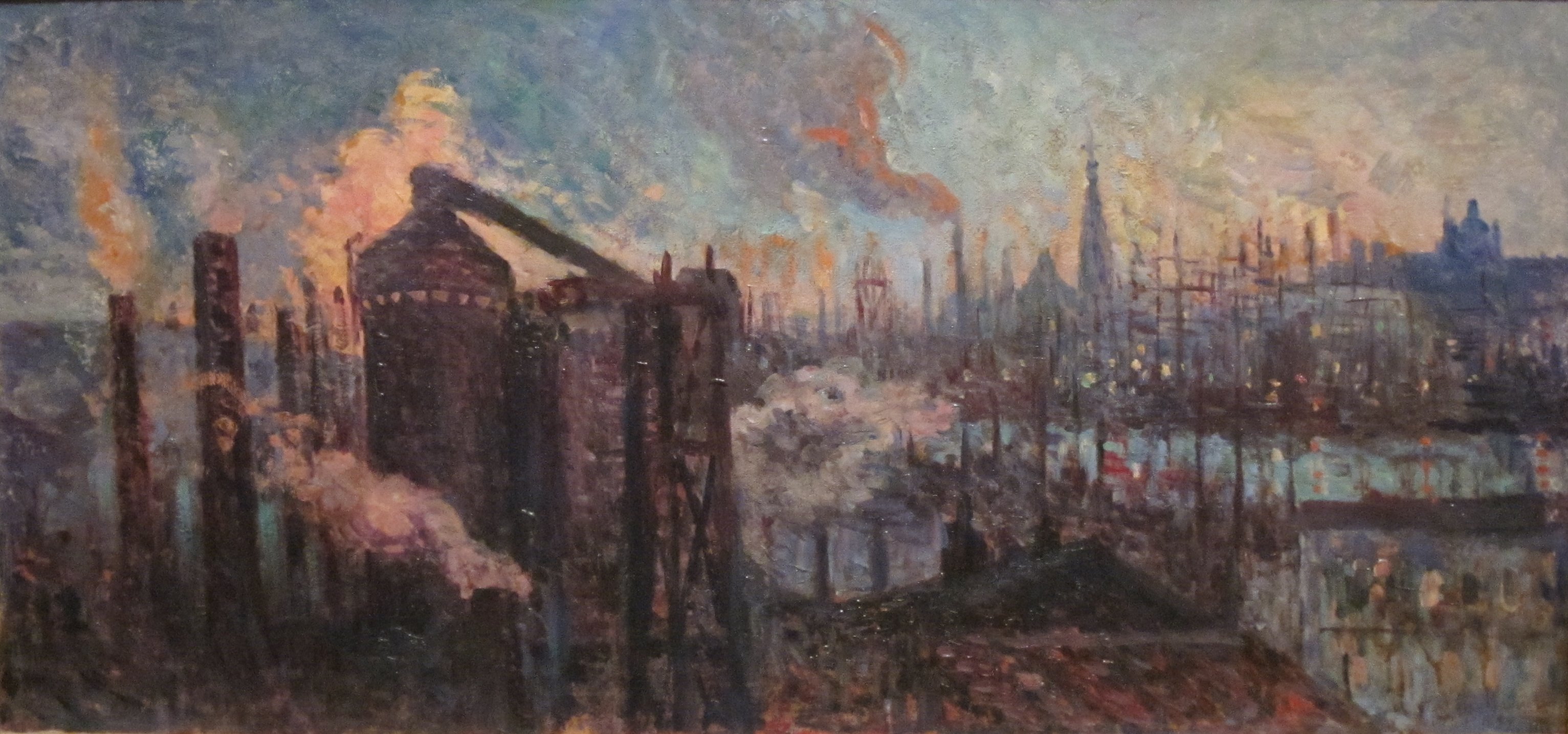This wide, rectangular painting depicts an expansive industrial landscape with a strikingly detailed scene. On the left side, there are several dark brown industrial buildings and apparatuses, emitting white smoke that billows across. These buildings are depicted in shades of bluish-gray and black, accentuating the gritty, industrial atmosphere. The sky above them is a dark blue, tinged with smoke and a red haze. As the eye moves towards the center and right side of the painting, the sky lightens to a gradient of lighter blue, fading almost to white. 

In the middle right, a serene, light blue, reflective body of water contrasts sharply with the industrial left. Behind this body of water, a city skyline emerges with several buildings, one of which has a prominent spire topped with a cross, suggesting it might be a church. The distant buildings are smaller, creating a sense of depth and distance. The perspective appears to be from a high vantage point, adding to the grandeur of the scene.

The painting boasts a color palette rich in light and dark blues, with accents of dark reds, oranges, and maroons. This palette enhances the overall atmospheric effect, blending industrial starkness with the nuances of an impressionistic style—evident in the visible individual brush strokes. The sky, loaded with both natural hues and industrial elements, features the sun in the upper right corner, adding a touch of warmth to the ostensibly dark scene.